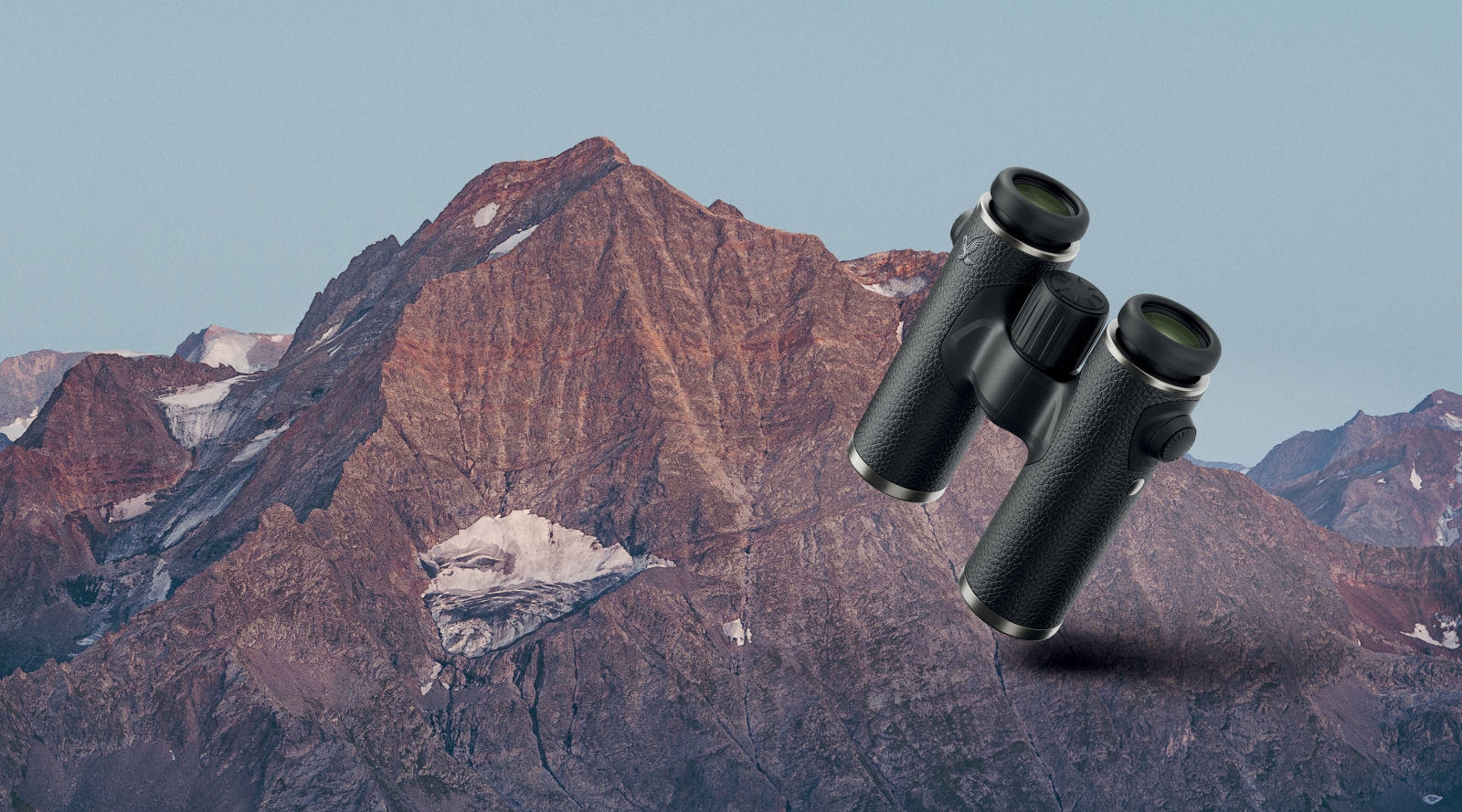In the foreground of the image, a pair of black binoculars with silver accents at the end of their lenses is prominently featured. The binoculars appear almost superimposed onto the background, creating an illusion that they are touching or right next to the mountain behind them. The mountain, predominantly reddish-brown with areas of grayish-blue shading and patches of white, forms the centerpiece of a rugged, rocky mountain range. The sky above is a clear, light blue with no clouds, highlighting the expansive outdoor setting. This atmospheric perspective is enhanced by multiple mountains visible in the distance on either side, adding depth to the scene. An intriguing detail is the shadow cast by the binoculars onto the mountain, reinforcing their presence in the photograph despite their seemingly suspended position.